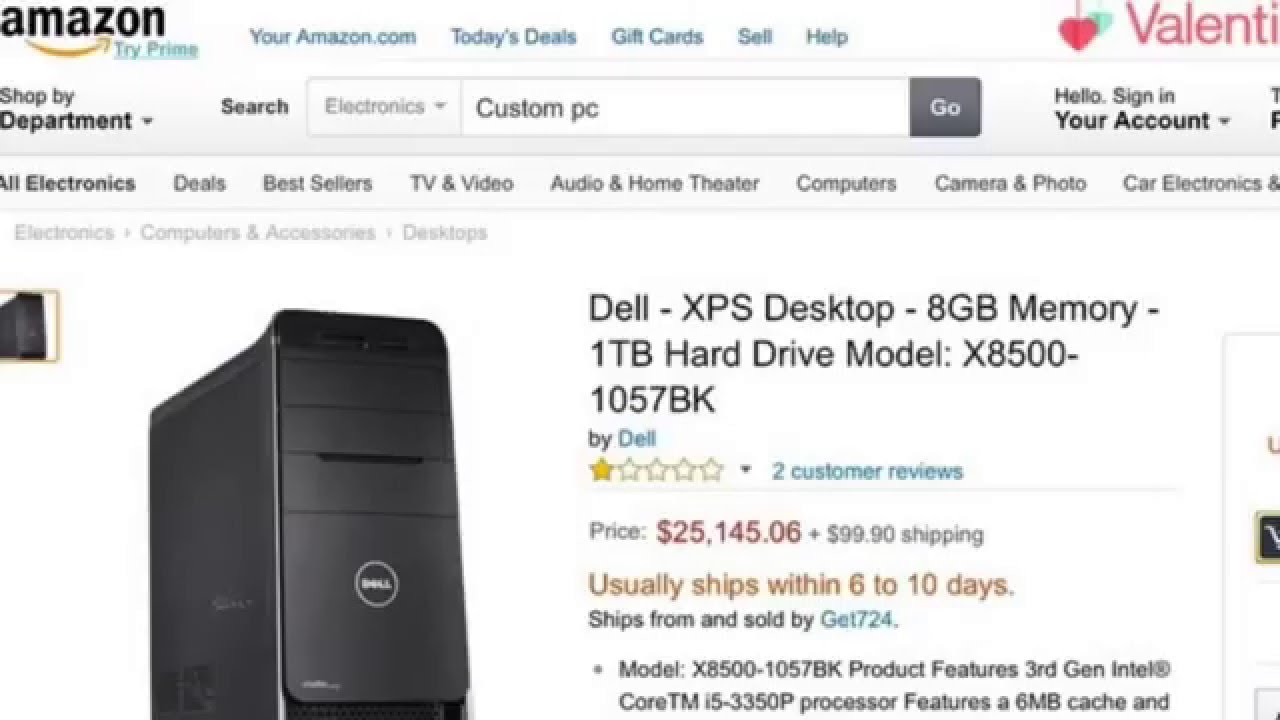Screenshot of Amazon Website: Dell XPS Desktop Listing

The screenshot captures a section of the Amazon website, prominently displaying a product listing for a Dell XPS desktop. The user, who does not have an Amazon Prime account as inferred from the "Try Prime" disclaimer, has searched for "custom PC" in the search bar. Among the search results is a Dell XPS desktop model X8500-1057BK, identified by its 8GB memory and a substantial 1TB hard drive.

**Product Details:**
- **Brand**: Dell
- **Model**: X8500-1057BK
- **Memory**: 8GB
- **Storage**: 1TB Hard Drive
- **Processor**: Third-Generation Intel Core TM i5-3350P with a 6MB cache
- **Color**: Black
- **Rating**: 1 out of 5 stars
- **Price**: Approximately $25,000
- **Shipping**: $99 fee
- **Availability**: Usually ships within 6 to 10 days
- **Seller**: Get724

Overall, this detailed product listing shows an expensive and low-rated desktop computer available on Amazon, highlighting specific features and shipping information.